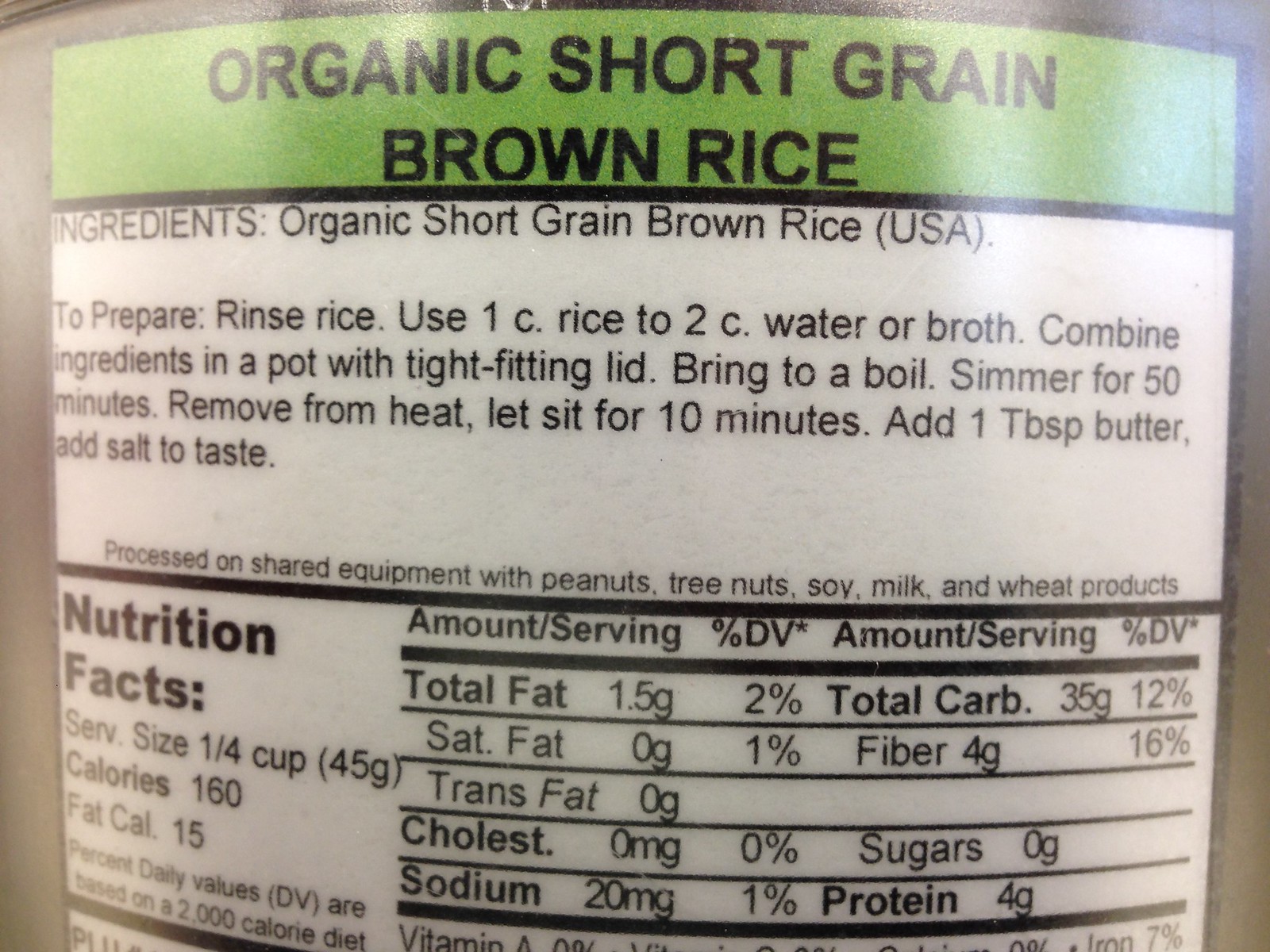The image depicts the back of a package of organic short-grain brown rice. At the top of the label, against a green background, it prominently displays "Organic Short Grain Brown Rice" in black capital letters. Below this, the sole ingredient is listed as "Organic Short Grain Brown Rice (USA)." Detailed preparation instructions follow in black text on a white background: rinse the rice, use one cup of rice to two cups of water or broth, combine ingredients in a pot with a tight-fitting lid, bring to a boil, then simmer for 50 minutes. After simmering, remove from heat and let it sit for 10 minutes. Add one tablespoon of butter and salt to taste. A warning notes that the product is processed on shared equipment with peanuts, tree nuts, soy, milk, and wheat products. The nutrition facts indicate a serving size of one-fourth cup, which provides 160 calories (15 from fat), 1.5 grams of total fat, 20 milligrams of sodium, 35 grams of total carbohydrates, and 4 grams of protein.